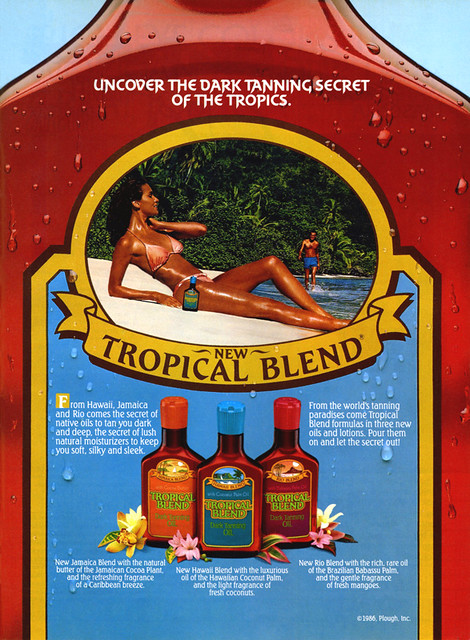This advertisement for New Tropical Blend tanning lotion features a vibrant and detailed layout. At the top of the blue bottle, outlined with a yellow border, is a prominent slogan in white text: "Uncover the dark tanning secret of the tropics." Below this, an image within a white-outlined circle showcases a sun-kissed woman in a pink bikini, lying on a towel by the water, with a bottle of the tanning lotion next to her. In the background, a man in blue swim shorts and a tropical treeline enhance the beachy ambiance. The bottle itself has a reddish-burgundy hue with water droplet patterns and features three different shades of the lotion depicted below the main image. These lotions, each with distinct colored caps—orange, blue, and red—are highlighted against a dark tanny-red background. The label includes small white text and a year, possibly 1956 or 1966, making it a nostalgic yet vibrant visual representation of the tanning product.